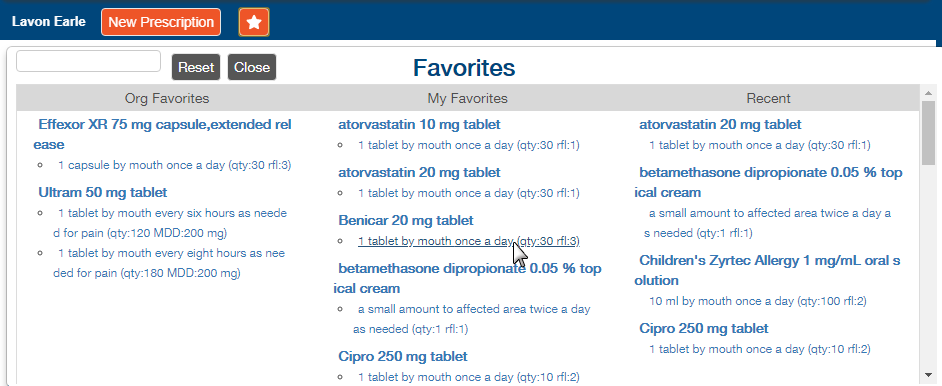Screenshot Description:

At the top of the screenshot, there is a blue bar spanning the width of the image. On the left-hand side of this blue bar, there is white text displaying the name "Lavon Earle". To the right, an orange button with white text reads "New Prescription," and a smaller orange button with a white star icon is also present. The rest of the top bar continues in blue.

Below the blue bar, the main section of the screenshot features a white background. At the top, there is a white search bar accompanied by two gray buttons: one labeled "Reset" and the other "Close," both in white text. Centrally placed below the search bar, in bluish-purple text, is the word "Favorites."

Further down, a gray bar contains the section headers. In black text, the left segment reads "Org Favorites," the center segment says "My Favorites," and the right segment shows "Recent."

The central white background below these headers lists various medications along with their dosage instructions. The first list contains two medications, the second has five, and the third holds four. Among these, the cursor highlights an instruction that reads "One Tablet per Mouth, Once Daily." On the far right of the screenshot, there is a vertical scrollbar for navigating through the page.